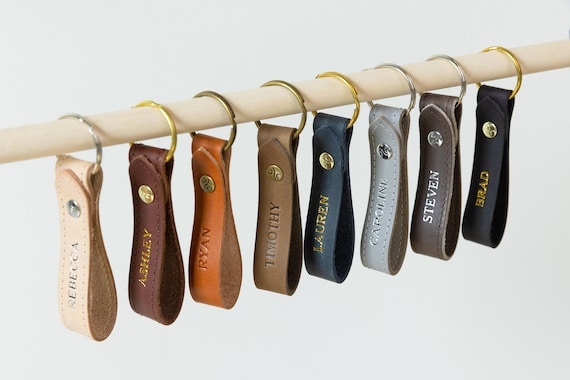The image is a professionally photographed close-up of leather keychains displayed on a brown wooden dowel against a clear or white background. The dowel runs horizontally across the picture, with eight leather keychains hanging from it. Each keychain is looped through a silver or gold key ring, secured by a matching silver or gold button. The dangling leather straps vary in color and each one is personalized with a name inscribed in metallic hues. From left to right, the colors and names are as follows: a very light tan one inscribed with "Rebecca," a dark brown one with "Ashley," a tan one with "Ryan," a lighter brown one with "Timothy," a dark blue one with "Lauren," a gray one with "Carolyn," a dark grayish brown one with "Stephen," and a black one with "Brad." The varying hues and metallic accents give each keychain a unique, customized appearance.